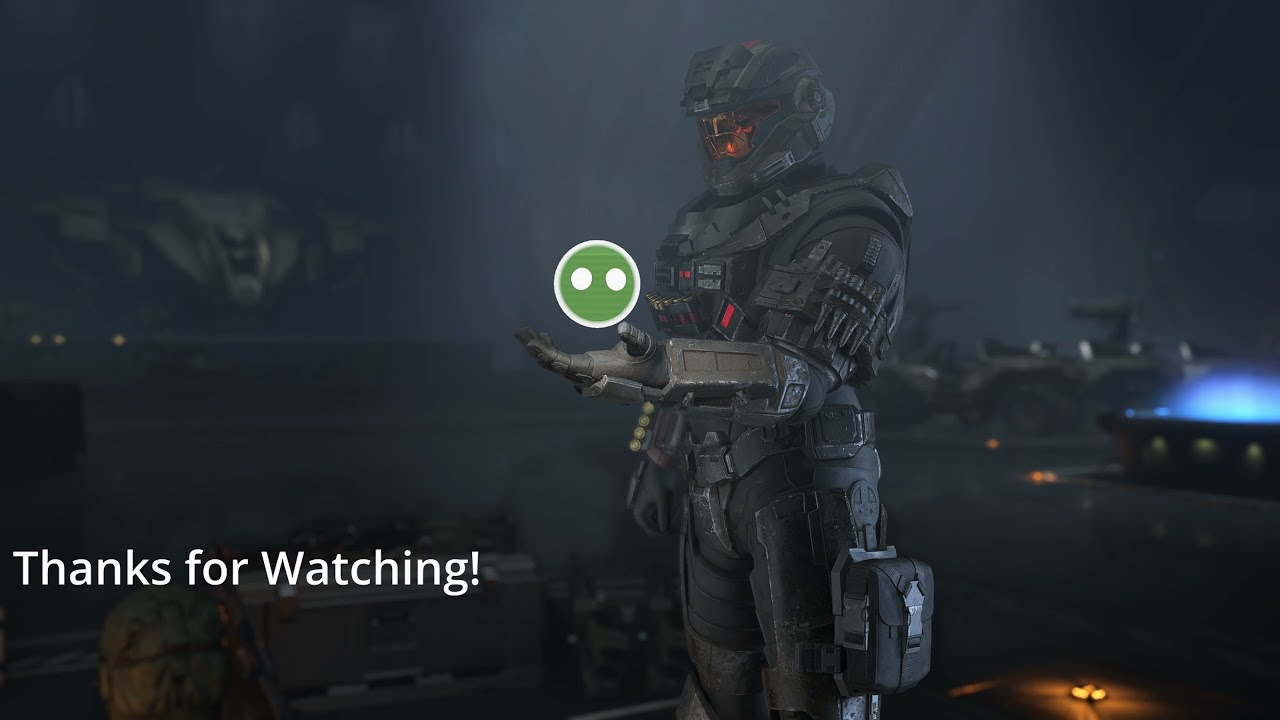In this high-definition still from a video game stream, a heavily armored soldier stands out prominently in the center of a dark, futuristic scene. Clad in robust, chunky gray armor with a distinctive burnt orange face guard, the character's appearance resembles a robot due to the sci-fi design elements and the numerous buttons and gizmos adorning the suit. The soldier is shown from the knees up, facing to the left, with their right hand resting by their side and their left arm extended, palm upwards as if offering or receiving something. 

Suspended just above the open palm is a green circle with white eyes, encased in a white border, adding a surreal touch to the otherwise photorealistic animation. This animated feature starkly contrasts with the realistic military aesthetic of the scene. 

In the dimly lit background, a futuristic fighter jet appears to be either landing or parked, alongside several other blurred military vehicles, creating a hazy, shadowy ambiance. The entire image is framed as if displayed on a large HD screen, typical of a gaming podcast or Twitch stream. To the lower left, white text reads, "Thanks for watching!" adding a friendly sign-off to this intense scene.